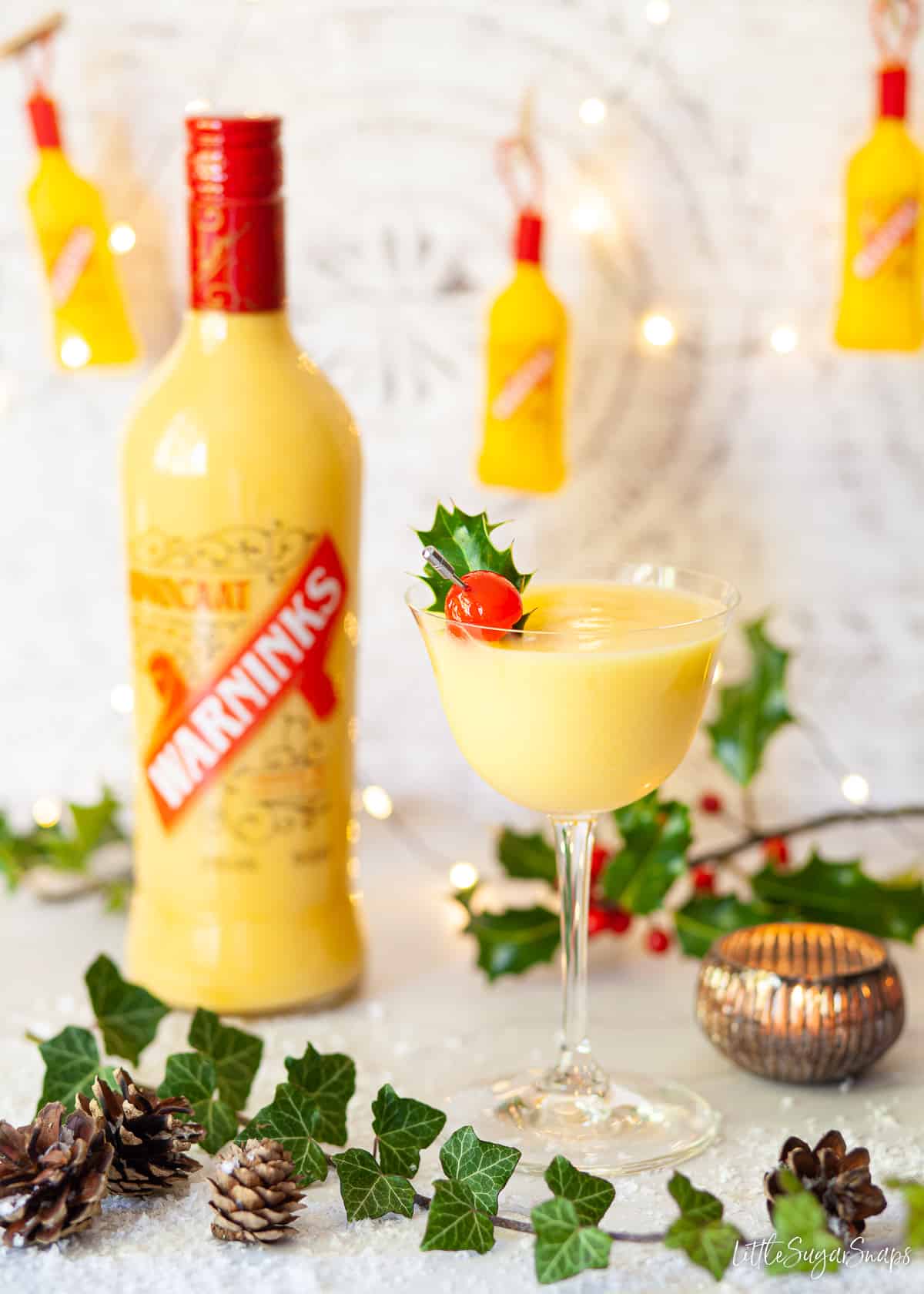This photo captures a festive holiday scene featuring a creamy eggnog cocktail in a crystal glass, prominently displayed against a backdrop of Christmas decorations. The cocktail itself is a thick, yellowish-white liquid, garnished with a cherry and a sprig of holly, lending it a seasonal touch. The surrounding decor includes green and brown tinsel, red berries, holly leaves, pine cones dusted with faux snow, and twinkling Christmas lights against a muted white wall.

In the foreground, a bottle of the yellowish liquor with a red cap is shown, branded as "WARNINKS." This distinctive bottle features a red label with white text and is matched by three similarly branded bottles hanging on hooks in the background. Additionally, a golden candle holder with a lit candle and cranberries among the holly enhance the holiday atmosphere. The scene evokes a warm, inviting Christmas setting, perfect for festive celebrations.